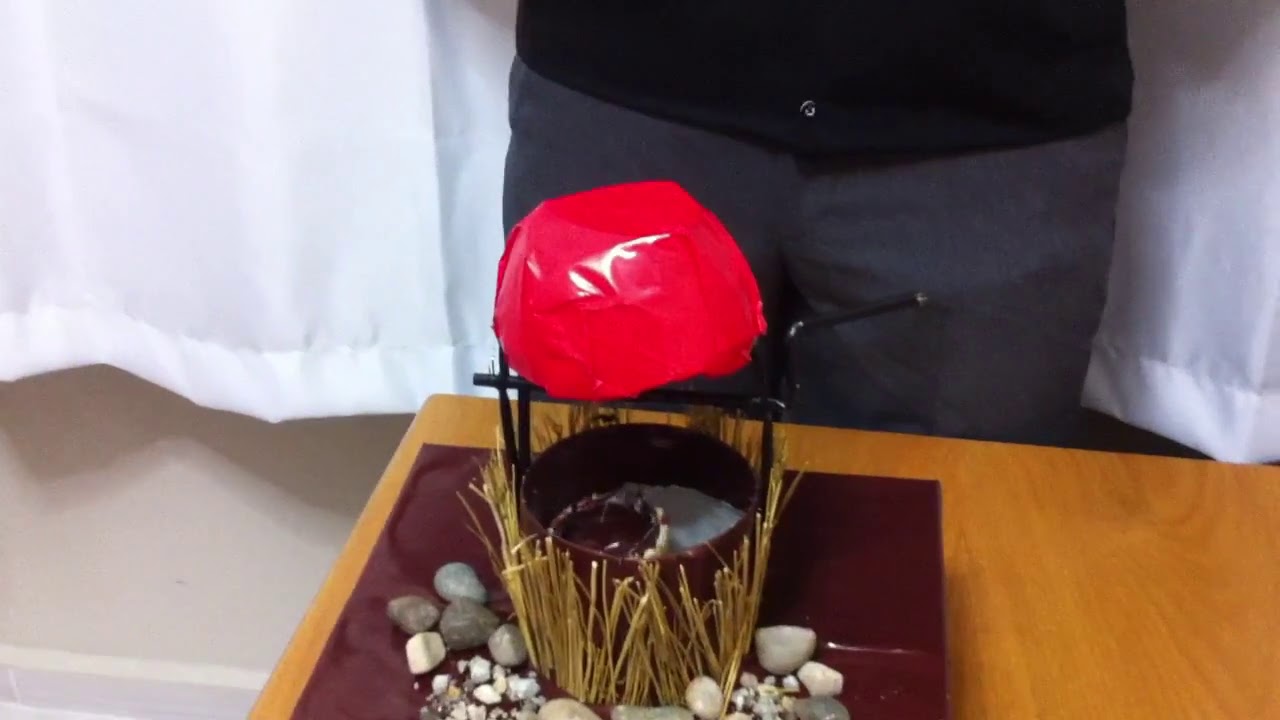This photograph showcases an intricate and somewhat confusing diorama resembling a miniature well, placed centrally on a brown wooden table. The centerpiece of this diorama is a small, circular pot, which appears to be a candle holder with a shiny red, cherry-colored dome acting as its roof. The pot is surrounded by scattered, shiny gray stones and adorned with light brown, hay-like straws, which seem glued to its exterior. A black metal frame with a handle and railings is visible, suggesting structural support for the dome, possibly hinting at a well-like design. Surrounding this setup is a square piece of purple or mauve material, enhancing the visual complexity of the display. In the background, a person is partially visible, dressed in dark gray pants and a black cardigan, standing against a white wall with white curtains. The enigmatic setup and the unusual combination of materials make the object's purpose hard to discern, evoking curiosity and interest.